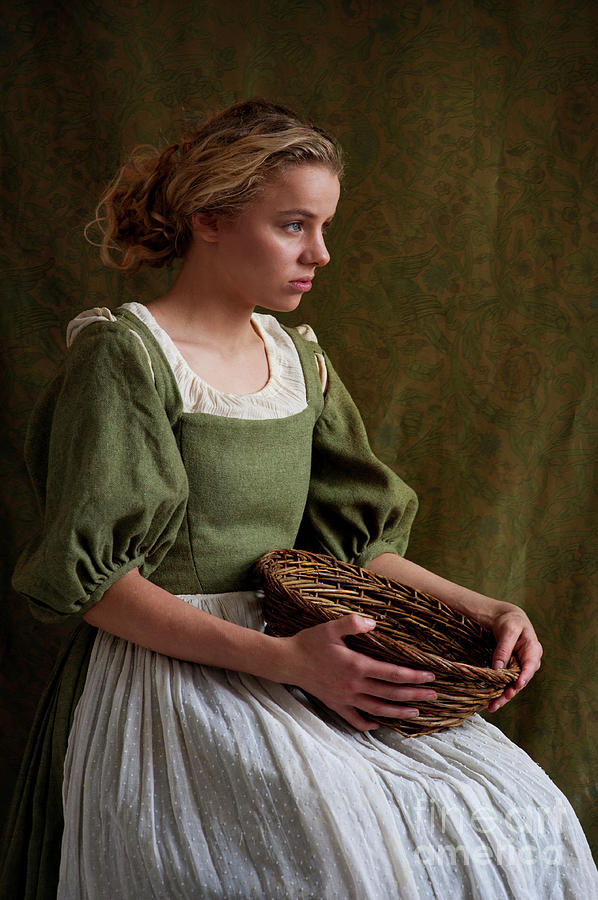The image depicts a young woman with blonde, curly hair tied back and blue eyes, seated and gazing towards the right. She wears an old-fashioned dress reminiscent of the early 1800s. The dress includes a white chemise underneath, visible beneath a green bodice or vest adorned with lace trim, and puffy sleeves that end at the elbows. Over the lower part of her dress, she wears a delicate white apron made of fine cotton. The backdrop is a green canvas that adds to the vintage aesthetic of the photograph. The woman holds an empty wicker basket on her lap, her expression appearing serious or contemplative. The image is marked "Fine Art America" in the lower right corner.